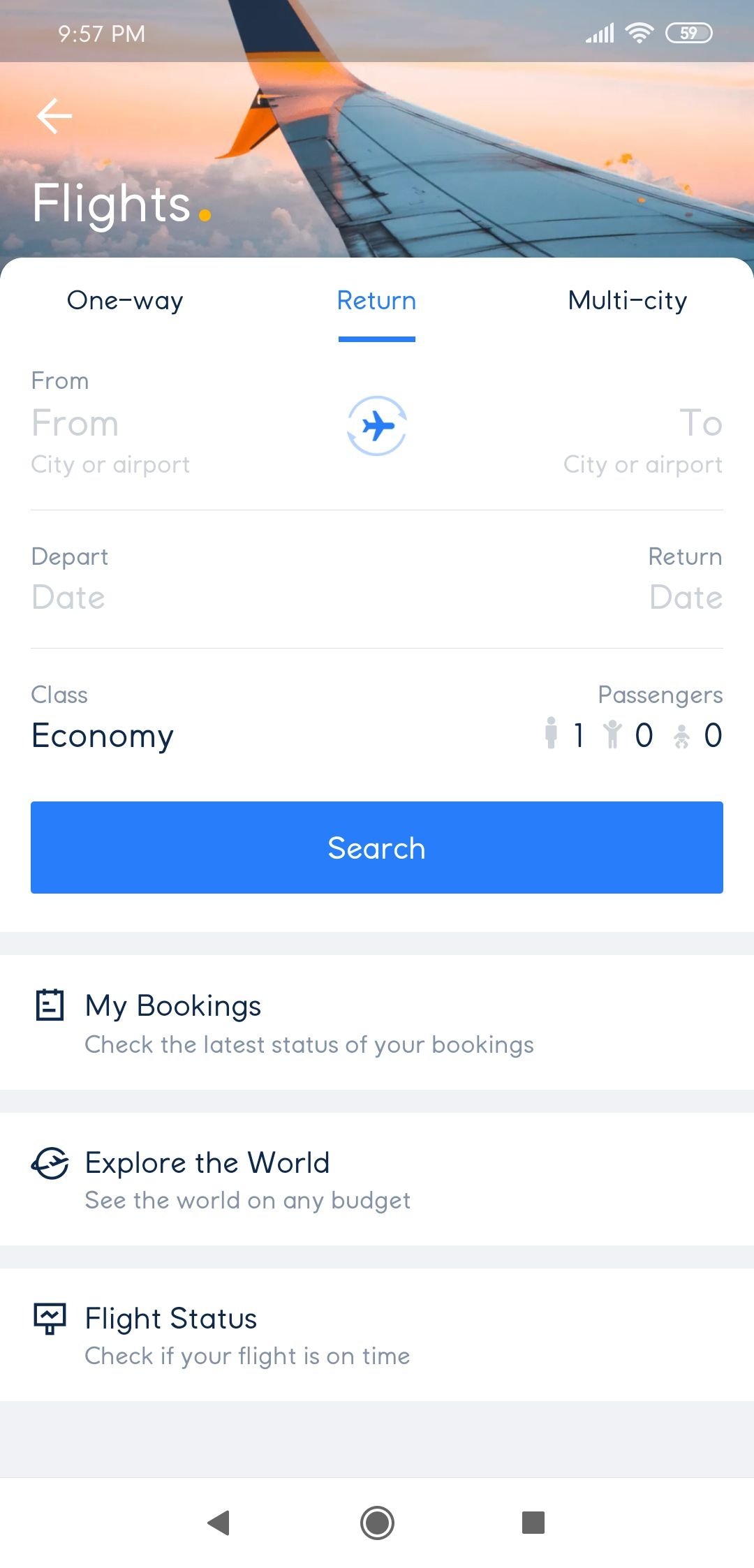A detailed screenshot is shown from an Android phone featuring the Google Flights application. The top part of the screen indicates it is 9:57 PM, with full mobile data connectivity (all 5 bars) and strong Wi-Fi connectivity (4 bars). The battery level is at 59%. The main menu is labeled "Flights," and the interface displays a vibrant image of an airplane wing captured from within the plane during a sunset, soaring above a bed of clouds.

Under the "Flights" label, the user has selected "Return" from a list that includes options like "One way" and "Multi-city." The fields for "From" (city or airport) and "To" (city or airport) are empty, as are the "Depart date" and "Return date" fields. The chosen travel class is "Economy," and one passenger is indicated. Below these options, there are buttons for "Search," "My bookings," "Explore the world," and "Flight status." The "My bookings" section advises users to "Check the latest status of your bookings," while "Explore the world" encourages users to "See the world on any budget." The "Flight status" section prompts users to "Check if your flight is on time."

At the very bottom of the screen, the three standard Android navigation buttons are visible: the "Back" button, the "Home" button (in the middle), and the "Recent apps" button.